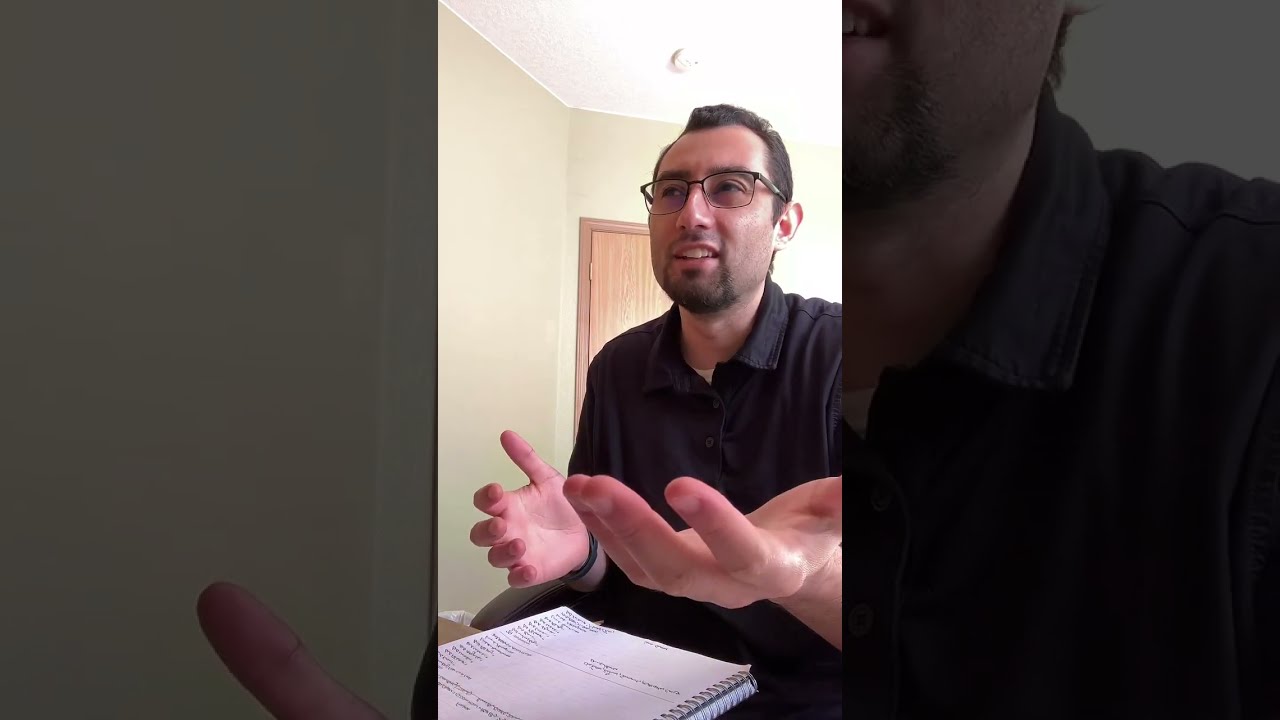The image is a triptych with the main picture in the center and mirrored, zoomed-in fragments on either side. The central picture is brightly lit and showcases a man who appears to be indoors, perhaps in an office setting. He has short, dark hair and is wearing roundish glasses that are slightly square at the bottom. He sports a black goatee and is dressed in a short-sleeve, collared shirt of a dark color, possibly black or deep purple.

In the central image, the man is looking slightly to his right with his palms facing upward, as though in the midst of explaining something. His facial expression is a mix of confusion and concentration, with his mouth slightly open and a hint of a smile. A spiral-bound notebook with some written notes lies open in front of him on a table.

The images on the left and right are darker and focus on specific portions of the central image. The left side zooms in on his pointer finger and a bit of his black shirt, along with the background wall. The right side highlights the upper portion of his black shirt and the lower half of his face.

Overall, the man appears to be engaged in a conversation, using his hands expressively to make a point, with the fragmented side images providing additional context to his gestures and posture.